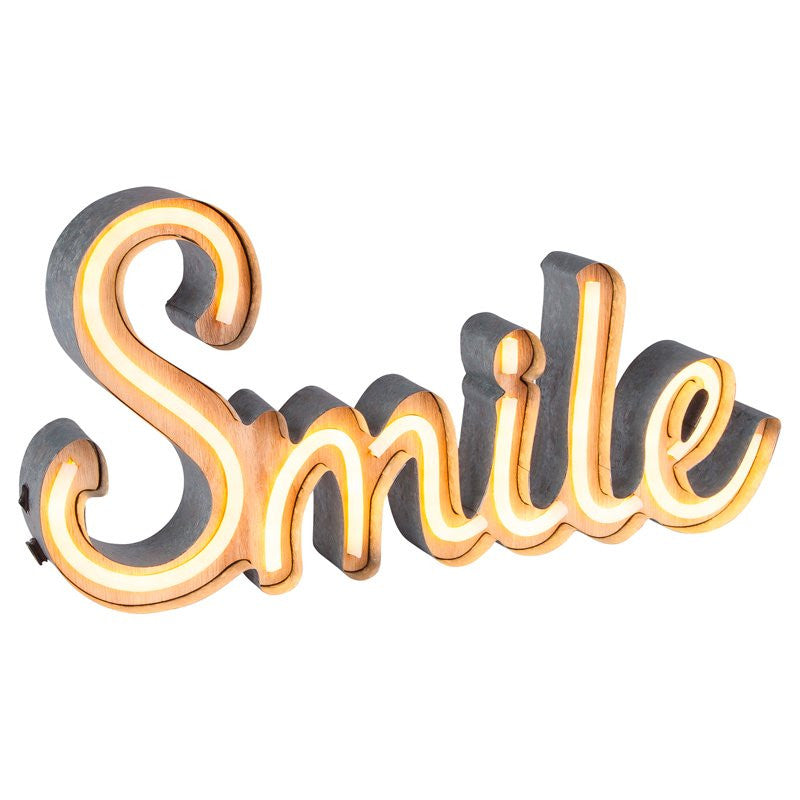This photograph captures a light-up neon sign that spells out the word "SMILE," elegantly crafted in a script-like, almost cursive font. Each letter is illuminated with a soft, glowing light that varies between gold and a hint of orange. The neon tubes are encased within a sleek, metallic structure, approximately 2-3 inches deep, that closely follows the contours of the letters. Surrounding the neon letters is a wooden frame, adding an artistic touch to the piece. The sign's on/off switch is subtly positioned on the lower curve of the 'S', consisting of a couple of small black knobs. The entire setup is placed against a stark white background, giving it a clean, product-like presentation, ideal for marketing purposes.